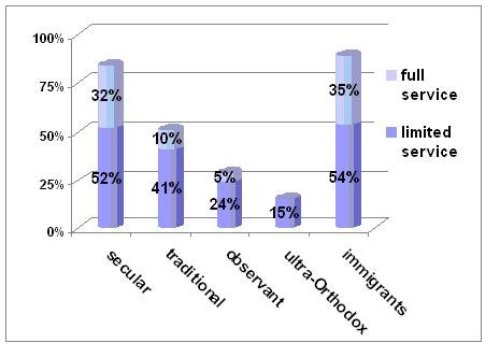The image depicts a detailed bar graph set against a plain white background that illustrates the distribution of full service and limited service across five distinct categories: Immigrants, Ultra-Orthodox, Observant, Traditional, and Secular. The x-axis classifies these five groups, while the y-axis ranges from 0% to 100%. Each category features a segmented bar representing the proportions of limited and full services offered. Dark blue segments indicate limited service, and light blue segments denote full service. Specifically, the Secular category shows 52% limited and 32% full service, Traditional shows 41% limited and 10% full, Observant shows 24% limited and 5% full, Ultra-Orthodox shows 15% limited service with no full service, and Immigrants show 54% limited and 35% full service. The overall visual presentation is framed within a square box, with category labels aligned below each corresponding bar.